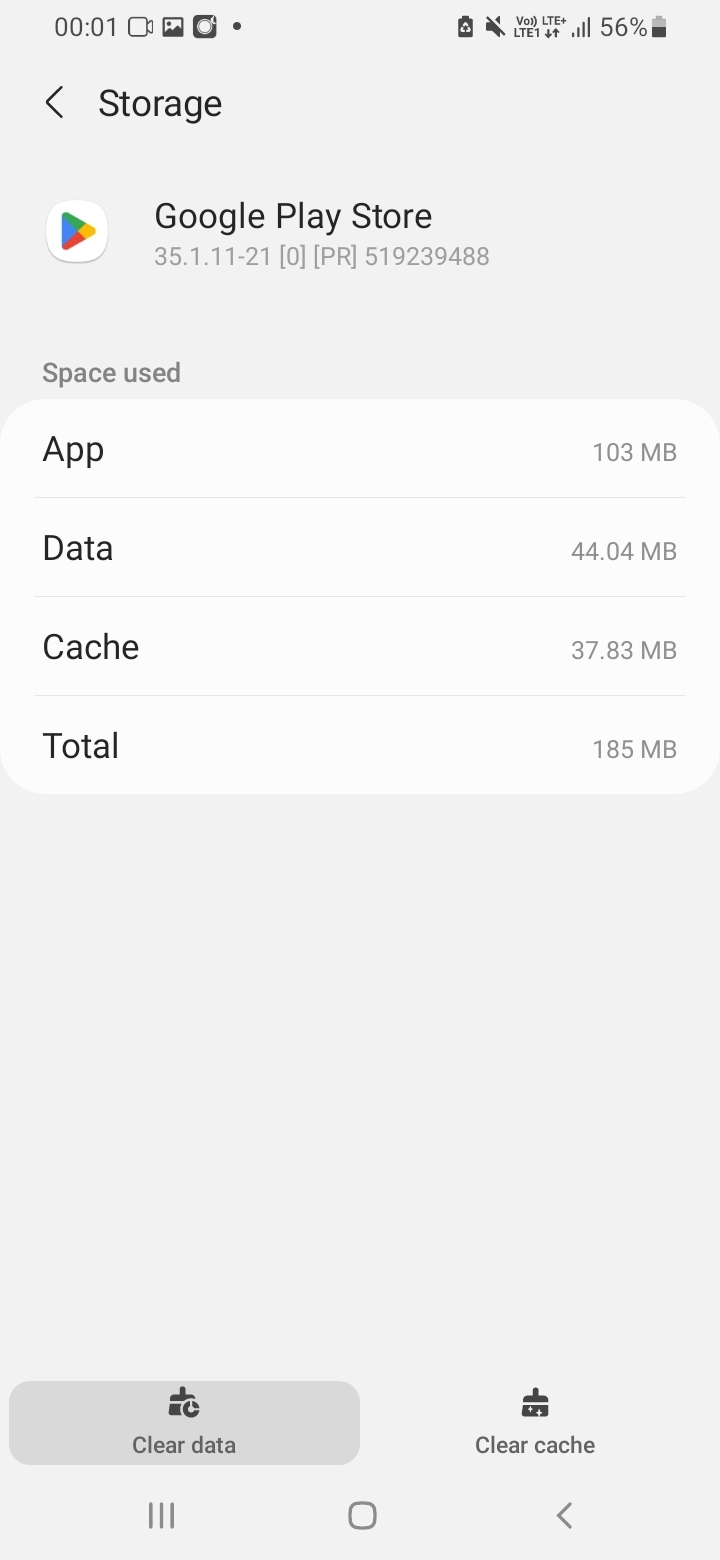This screenshot captured from a smartphone displays the Google Play Store information page within the device's storage settings. At the top of the page, a title bar reads "Storage" with a back button positioned on its left side. The version of the Google Play Store app is noted as 35.1.11-21.

Below the version information, the storage usage is broken down into four categories:
- App: 103 megabytes
- Data: 44 megabytes
- Cache: 37 megabytes
- Total: 185 megabytes

At the bottom of the page, there are two option buttons for managing the app's storage:

1. **Clear Data**: Represented with a circular graph icon.
2. **Clear Cache**: Represented with a paintbrush icon adorned with magic sparks.

Surrounding the app-specific information, the phone's system interface elements are visible, including the status bar at the top, showing the time and battery level, and navigation options at the bottom, such as the home button and the "Close All" command.